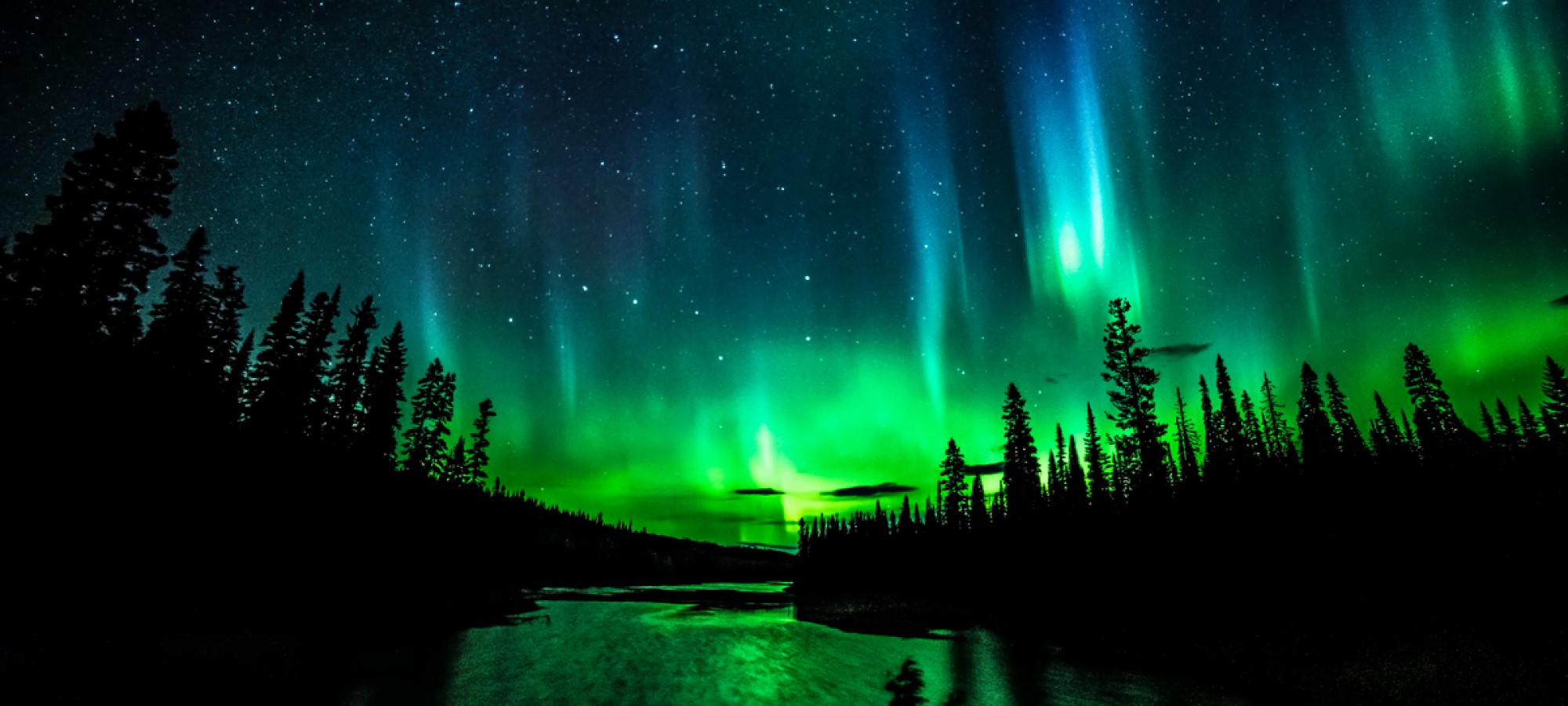This color photograph captures the mesmerizing beauty of the Northern Lights, or Aurora Borealis, in a nighttime nature scene. In the foreground, a wide river reflects the vivid greens of the Aurora, flanked by the black silhouettes of tall, skinny pine trees on either bank. The sky above dominates the image, adorned with a cascade of the Northern Lights in spectacular shades of green, lemon yellow, light blue, and streaks of white mingling with blurry clouds. On the left side, the sky is dotted with countless stars, adding a celestial sparkle to the scene. The dark navy blue and black hues of the night sky provide a striking contrast against the Aurora, which appears to be emanating from the horizon, almost giving the illusion of a UFO landing. This breathtaking photograph beautifully encapsulates the awe-inspiring natural phenomenon of the Northern Lights against a serene, starlit backdrop.